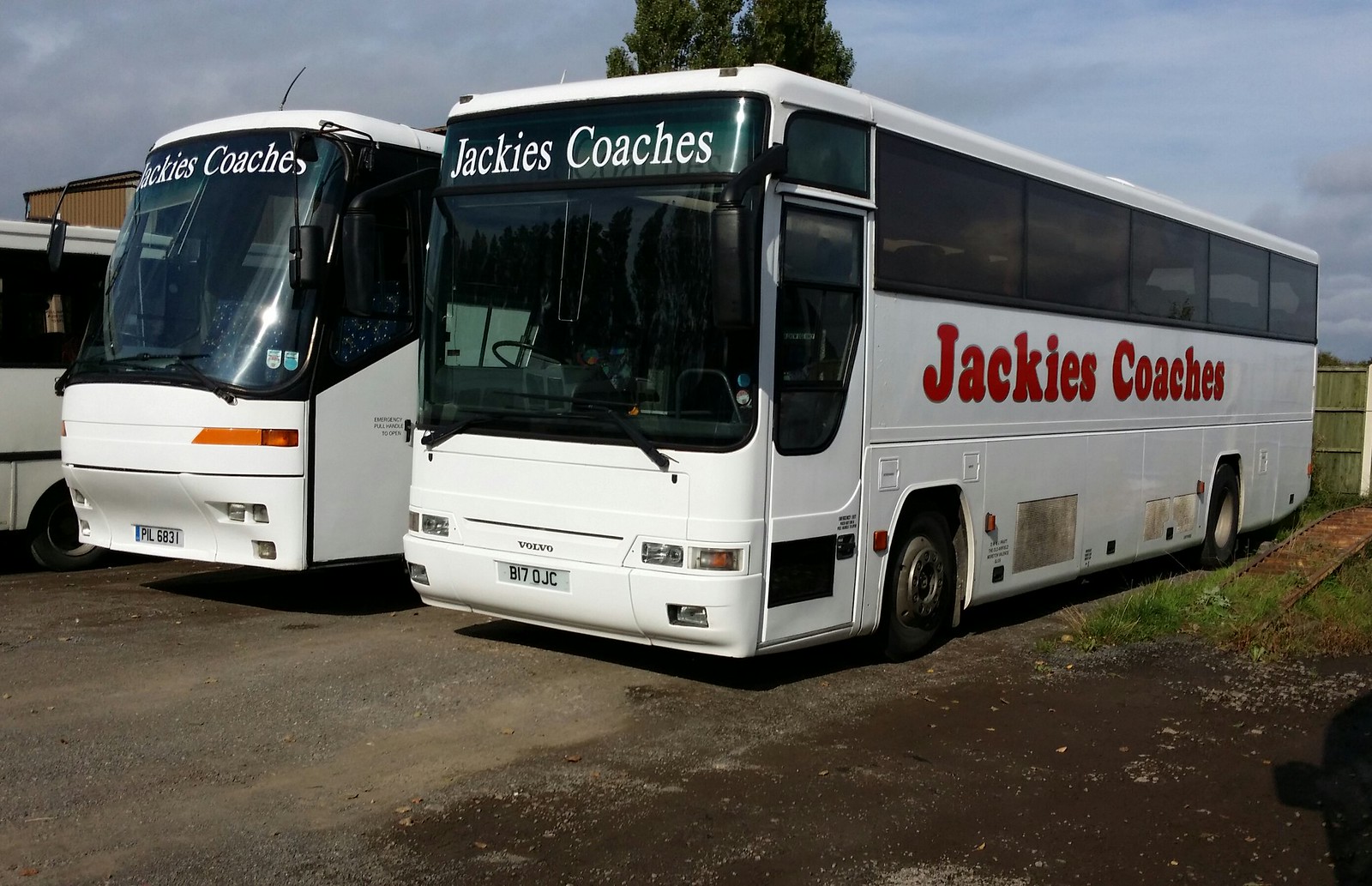This photograph captures a dirt lot where three large white buses are parked side by side. The buses, marked with red "Jackie's Coaches" lettering on their sides and white "Jackie's Coaches" text on the upper part of their windshields, appear to be tour buses. Although only two of the buses are fully visible, their license plates can be clearly read: B170JC on the right bus and PIL 6831 on the left bus. The photograph seems to be taken on a partly cloudy day, adding a neutral light to the scene. Surrounding the buses is a wooden fence, covered in green moss, which runs behind them. An old, rusted metal ramp extends near the buses, suggesting a service area that the buses might use. There's green grass growing by the ramp as well. To the right, part of a tree is visible, adding a touch of nature to the otherwise industrial setting. No people are present in the image, focusing the viewer’s attention on the buses and their surroundings.